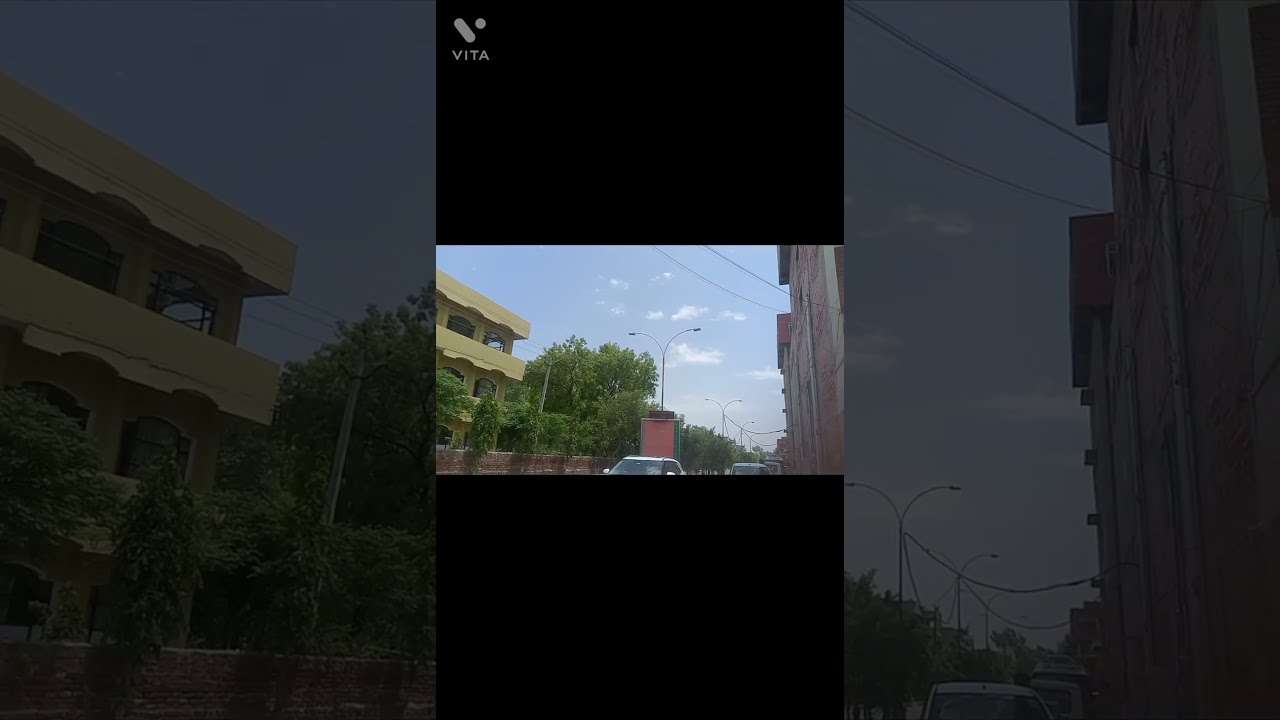The image is a detailed photograph of a streetscape, with an intriguing overlay effect. The primary photograph, slightly grayed out and blurred, spans from left to right and depicts a parking area along a side street, with a backdrop of green foliage and various brick buildings. Running through the middle of this large photo is a smaller, more vibrant version of the same image. This central photograph has substantial black borders at both the top and bottom, taking up roughly one-third of the overall image height. In the upper left corner of the central picture, the word "Vita" is displayed alongside a small gray line and dot.

The more vibrant central image showcases a yellow, multi-story building prominently on the left, surrounded by trees and a red brick wall. To the right, you can see multiple street lamps, power lines, and a row of brick buildings. Topping off the scene are a few street-parked cars visible near the bottom of the smaller photo. The composition creates a striking "picture within a picture" effect, magnifying the details of the central building and surrounding street while maintaining a border of the grayed-out, larger photograph that contextualizes the urban setting.